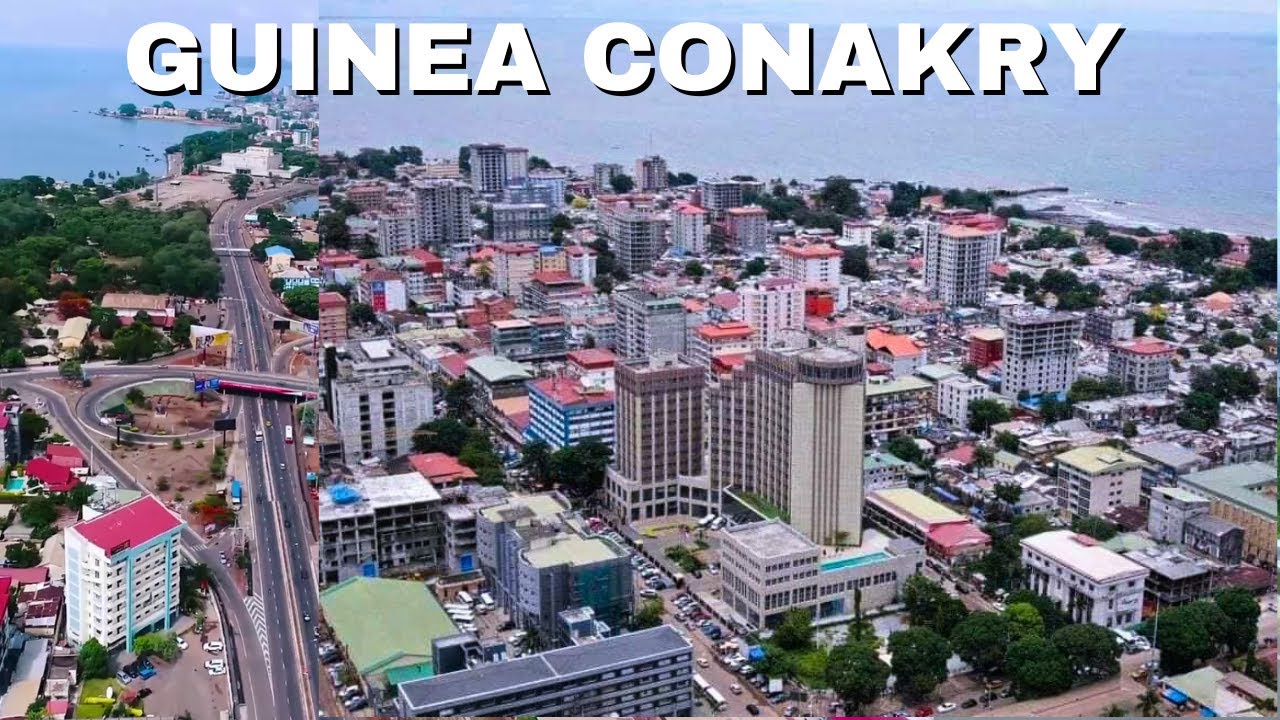This aerial image captures a densely inhabited coastal city identified by bold white text with a black drop shadow at the top reading "Guinea-Conakry." Prominent in the photo is a main road on the left side, featuring a roundabout or interchange with connecting ramps, which bends right to follow the coastline. The cityscape displays numerous tall buildings, likely reaching up to 20-25 floors, predominantly concrete structures that could be hotels or business offices. Smaller buildings are also visible, some under construction, indicating development. Several cars are parked around the buildings, and the city stretches out towards and partly into the ocean, creating a peninsula-like shape. The overall scene suggests a mix of residential and commercial areas, with a dense but organized urban layout.